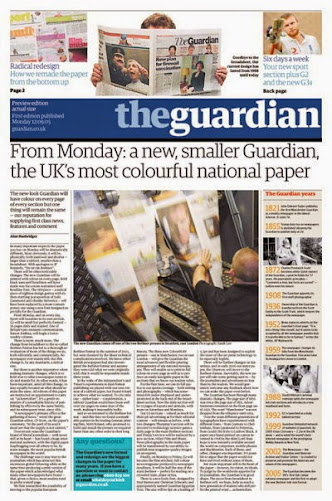In the photograph, we observe a newspaper-like article from "The Guardian." A blue banner prominently displays the title, "The Guardian," with "The" in light blue and "Guardian" in white. At the upper part of the image, a man with blonde hair is visibly engrossed in reading the paper, holding it open with both hands. To the right of this scene, text announces, "Six days, eight week. Your new sport section plus G2 and the new G3U." Adjacent to this, a lacrosse player is depicted, wearing a white jersey marked with the number two, sporting blonde hair and a blonde beard.

Above these elements, a large black banner proclaims, "From Monday, a new smaller Guardian. The UK's most colorful national paper." Another significant detail in the image is a bald man dressed in a black shirt with a watch, interacting with a touchscreen that displays various news articles.